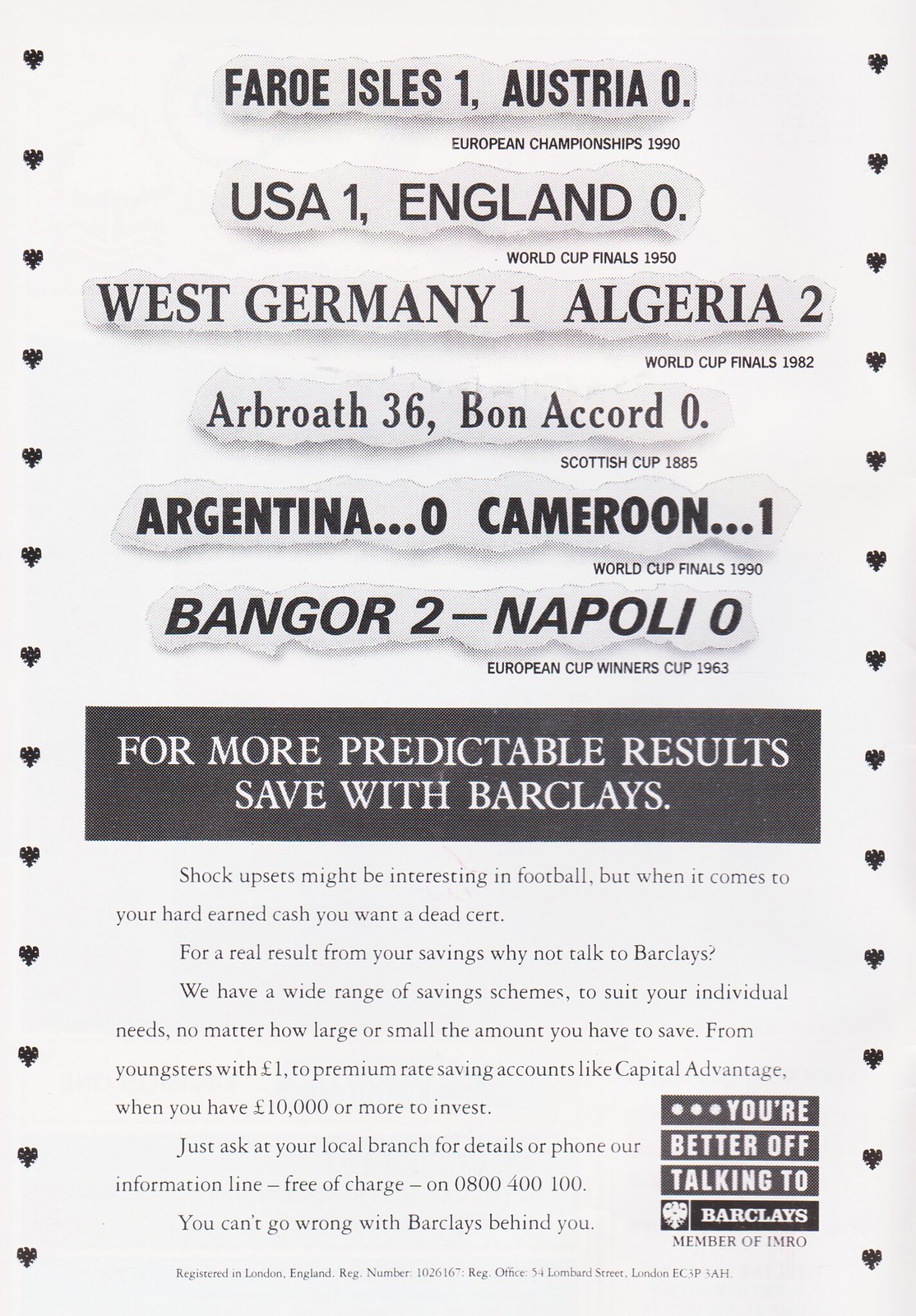This black-and-white poster features sports scores against a white background with black text. Along the vertical sides, there are rows of small black hearts. The main text details several notable soccer match outcomes, highlighting iconic moments in football history. The scores are listed as follows: Faroe Isles 1, Austria 0 during the European Championships 1990; USA 1, England 0 in the World Cup Finals 1950; West Germany 1, Algeria 2 in the World Cup Finals 1982; Arbroath 36, Bon Accord 0 in what appears to be a Scottish Cup match; Argentina 0, Cameroon 1 in the World Cup Finals 1990; and Bangor 2, Napoli 0 in the European Cup Winners' match of 1963. At the bottom, there is a promotional message from Barclays Bank, which reads, "For more predictable results, save with Barclays. Shock upsets might be interesting in football, but when it comes to your hard-earned cash, you want a dead cert."